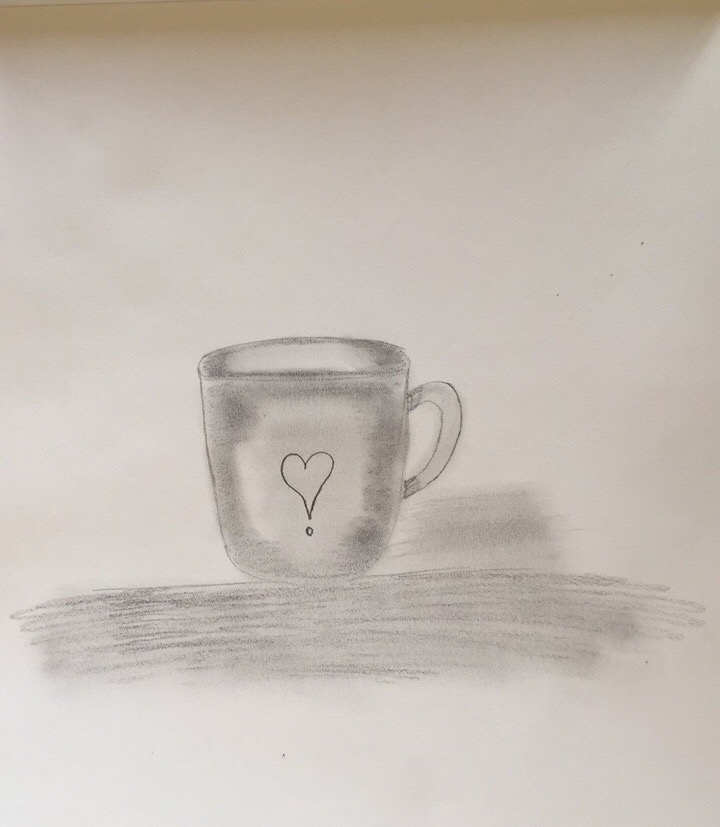This is a meticulously crafted pencil drawing on unbleached, natural white paper with subtle grayish undertones and hints of beige. The artwork features a ceramic-style coffee cup with a charming heart design in the center, accompanied by a small dot below the heart. The cup showcases intricate shading, giving it a realistic and solid appearance. The rim of the cup is notably thick, suggesting a sturdy construction. Despite its petite size, likely holding around six to eight ounces, the cup's handle is disproportionately small, seemingly allowing room for only a few fingers. Beneath the cup, a faint scribble symbolizes the surface or table on which the cup rests, adding a touch of context to the drawing.